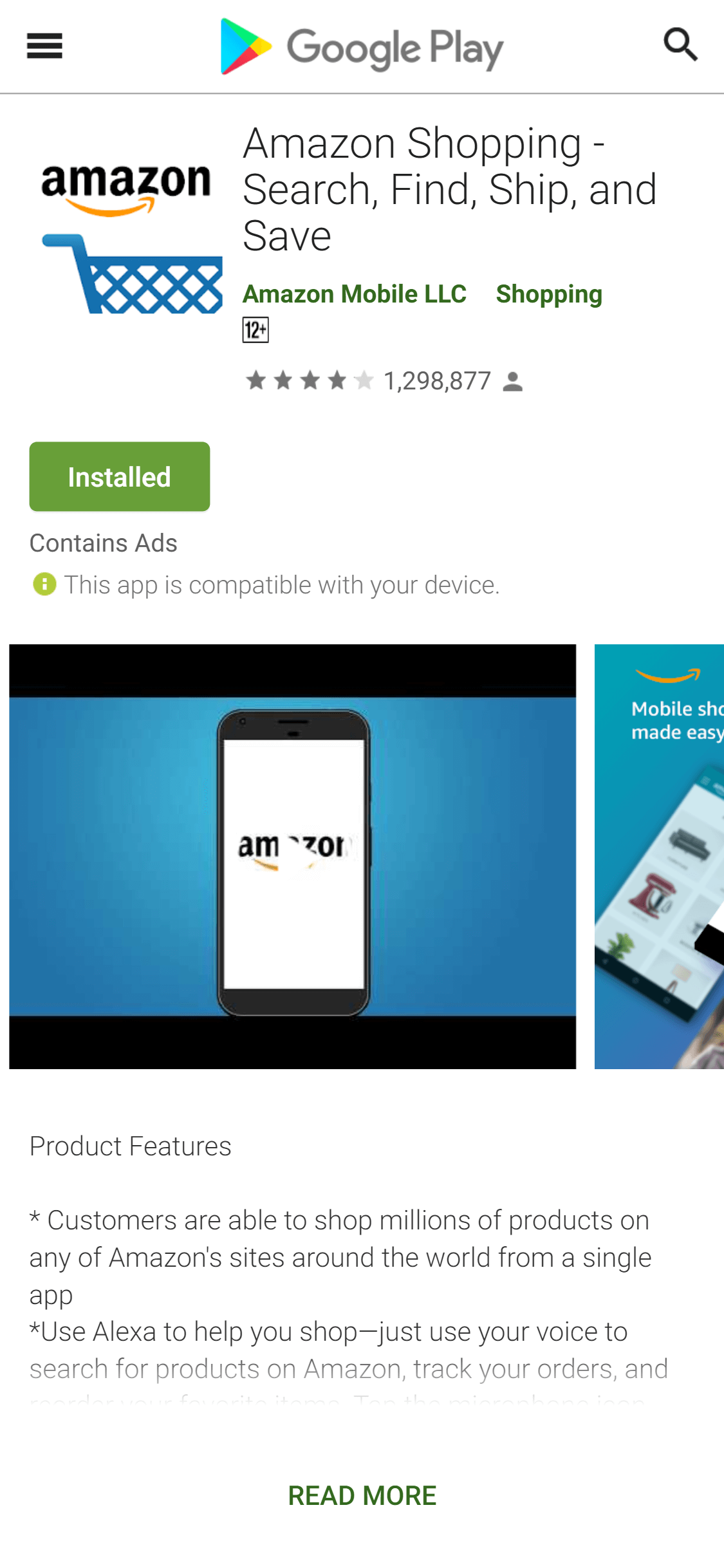This vertical screenshot, optimized for mobile viewing, showcases the Google Play Store's page for the "Amazon Shopping" app. At the top, the familiar Google Play logo is prominent, followed by the three horizontal bars on the left, indicating the menu. Below a gray dividing line, the app's title "Amazon Shopping: Search, Find, Ship, and Save" is displayed, developed by Amazon Mobile LLC. The app is suitable for users aged 12 and above and boasts an impressive rating of 4 out of 5 stars, based on 1,298,877 reviews.

An iconic Amazon logo is superimposed on a blue shopping cart graphic, positioned adjacent to a green rectangular button labeled "Installed." Directly beneath, it notes the presence of ads and confirms the app's compatibility with the user's device.

A video section follows, framed by black bars on the top and bottom, with a blue background featuring an image of a mobile phone and a play button, inviting users to watch a demonstration. Below the video, a brief outline of the app's product features is provided: customers can shop millions of products on Amazon's global sites from a single app, utilize Alexa for voice-activated searches, and track their orders. The section concludes with a "Read More" prompt for additional information.